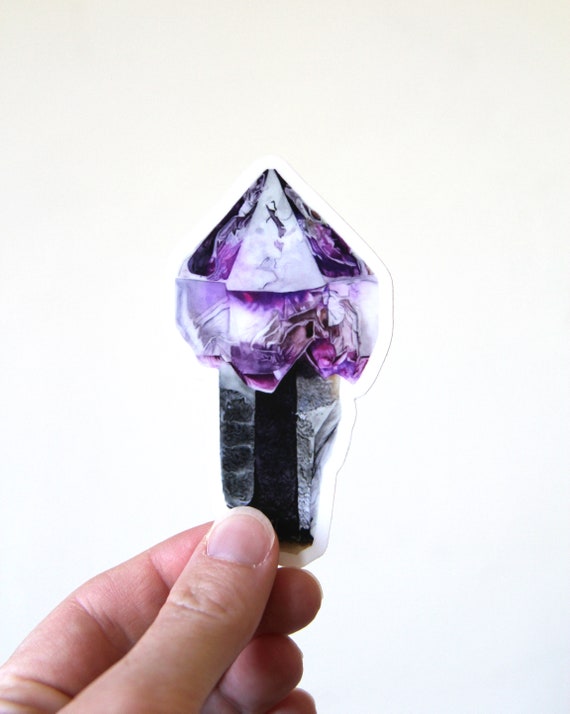This is a realistic vertical photograph with a predominantly white background that subtly transitions from a lighter shade in the top left to a slightly darker tone in the bottom right. Central to the image is an adult’s left hand, primarily showing the thumb and the tips of the index and middle fingers, delicately holding a detailed sticker. The sticker features an ornate depiction of an amethyst stone. The stone illustration has a multifaceted, jagged appearance, starting with a deep, vibrant purple at the top that gradually fades into lighter shades of purple toward the middle. The base of the stone is represented in black, resembling the color of shale. The intricate design of the sticker captures the reflective qualities of an actual gemstone, emphasizing its detailed and realistic presentation.